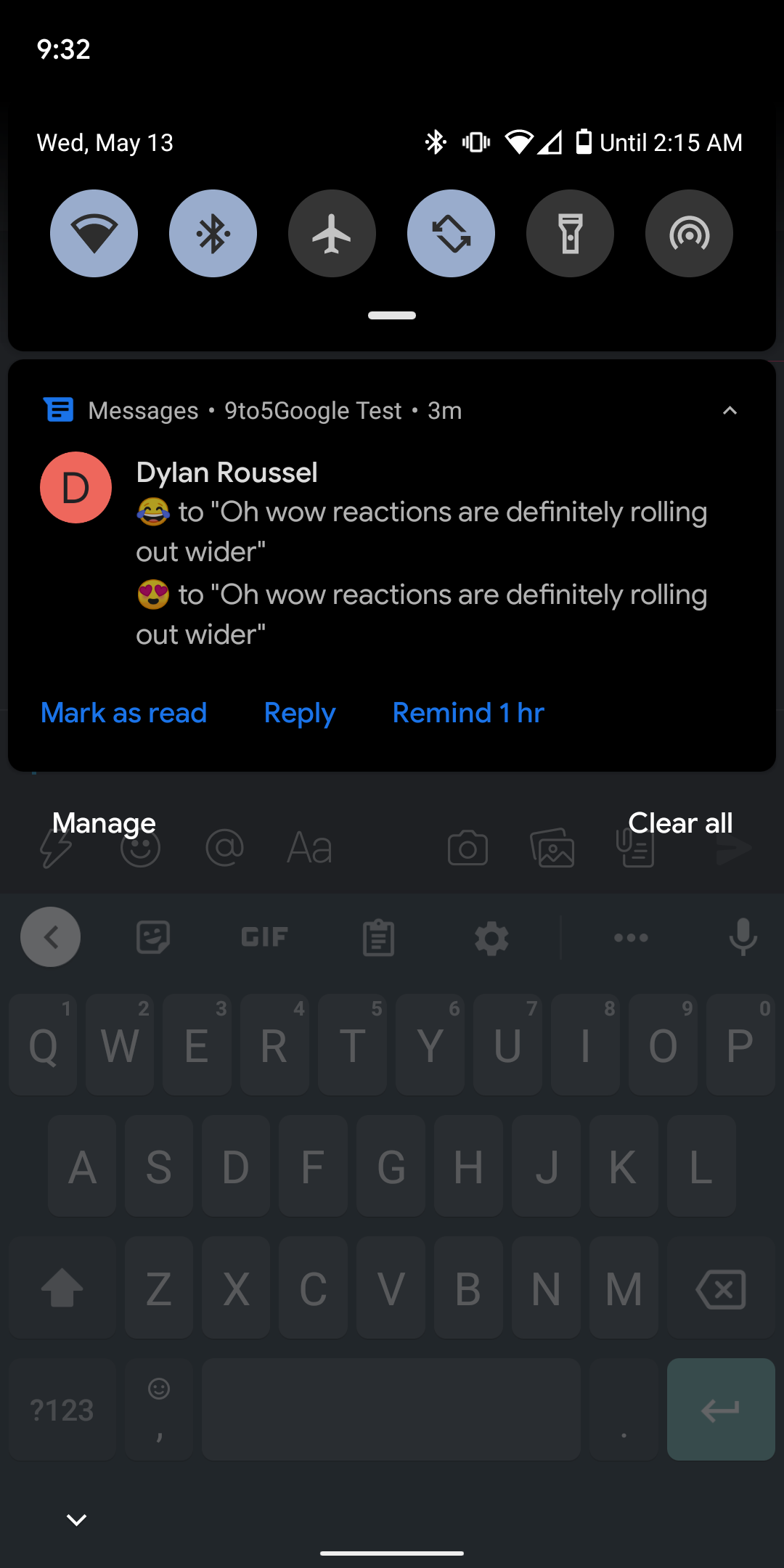A detailed screenshot of a mobile phone at 9:32 PM featuring a primarily black background with white text. At the top, the settings menu is visible, showcasing toggles for Wi-Fi, Bluetooth (active), airplane mode, portrait mode, flashlight, and location sharing (active) against a black background. Above these toggles, the date and time, "Wednesday, May 13th, 9:32 PM," are displayed. The screen also indicates an almost full Wi-Fi signal, a very low mobile data signal, and a nearly depleted battery.

Below the settings menu, the "Messages" app is open, showing a recent message from "9to5Google" received 3 minutes ago. The conversation is headed by a pink circle with the letter "D," identifying the contact as Dylan Russell. The text message contains laughing-crying emojis, indicating amusement: "😂" followed by the text, "Oh wow, reactions are definitely rolling out wider." Further down, a heart-eyes emoji "😍" accompanies the repeated message, "Oh wow, reactions are definitely rolling out wider." Options for "Mark as read," "Reply," and "Remind in 1 hour" are available in blue font at the bottom of the message.